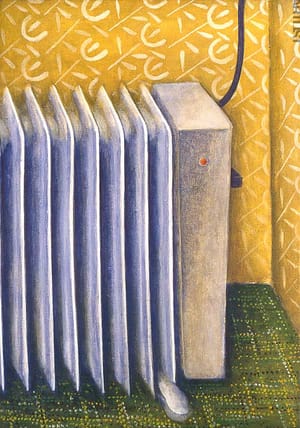The image is a detailed painted artwork depicting the corner of an old-fashioned room. The room features yellow and white patterned wallpaper with flowery motifs, adding to the outdated aesthetic. A prominently placed silver radiator sits on a green carpet with a checkered pattern incorporating yellow, black, and white squares. The radiator, made of chrome metallic material, has a black cord plugged into an unseen outlet and a non-illuminated red indicator light on its side. The overall setting is vibrant, with the bright gold hues of the wallpaper and the grass-green tones of the carpet contributing to its vivid portrayal.